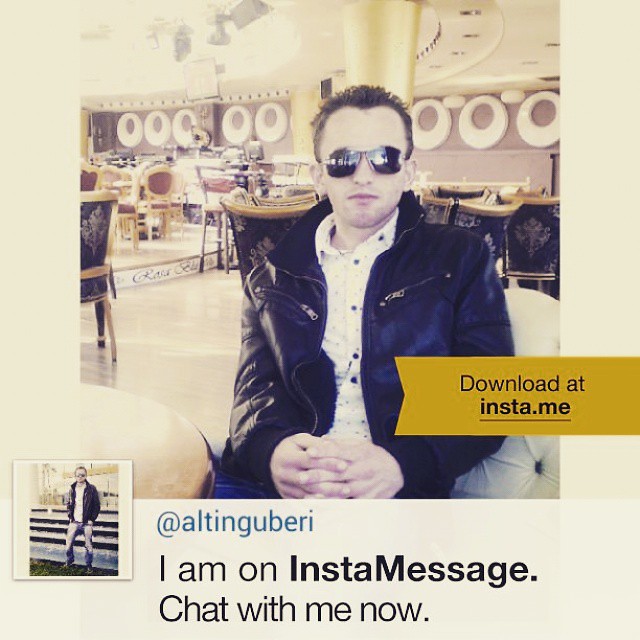In the image, a young adult man is seated in a dining room of a restaurant. He wears a black leather jacket over a white collared shirt with black buttons, and dark sunglasses, his short, spiky hair contributing to his stylish demeanor. His hands are clasped in his lap, and he looks directly at the camera. The dining room exudes elegance with its fancy chairs and ornate circular artwork on the walls. A gold-colored column stands prominently behind him. The image serves as an advertisement for his InstaMessage handle, @Altingubri, encouraging viewers to chat with him now. Alongside, in the cream-colored background, blue text reiterates his handle. A small, goldenrod banner on the photo promotes downloading Insta.me. Additionally, a smaller inset photo in the bottom left corner shows the same man standing in front of stairs, wearing the same outfit.